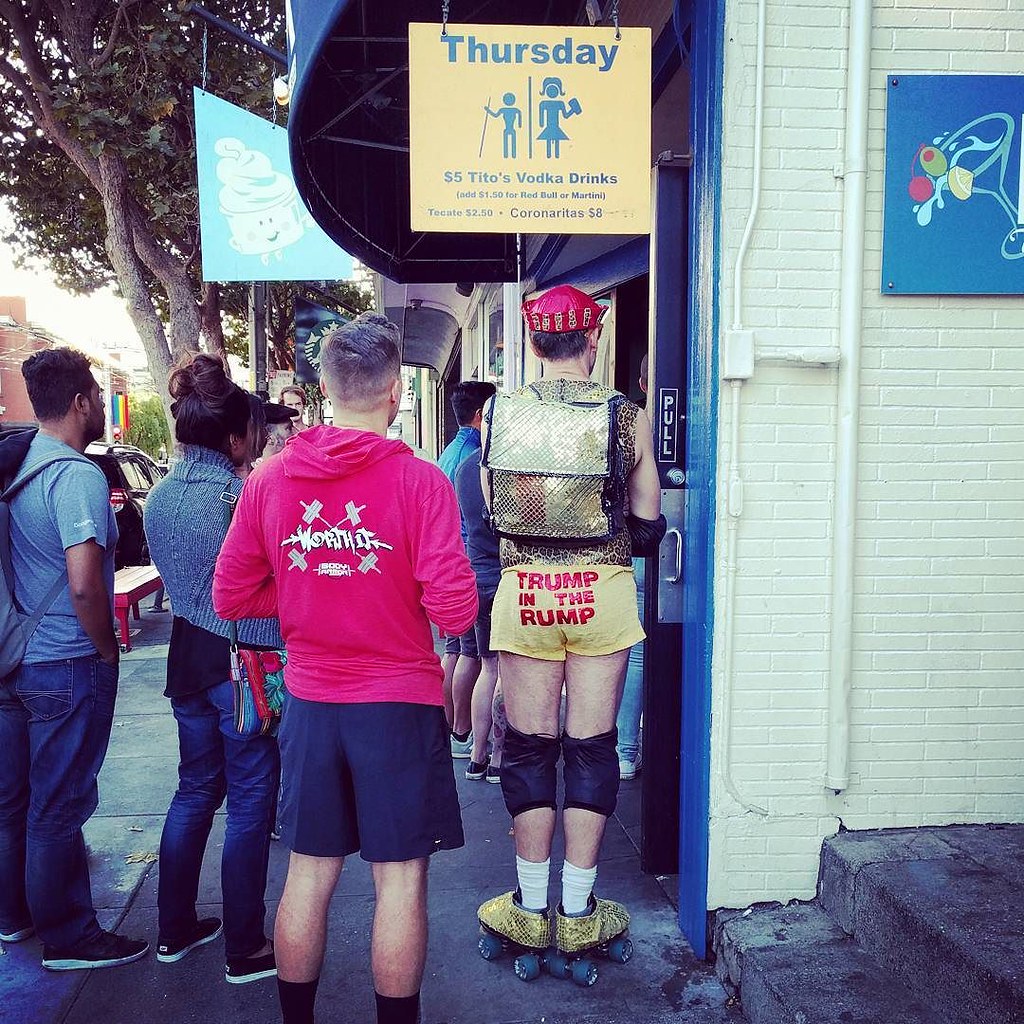On a clear day, outside what appears to be a bar with a white brick exterior and a blue entranceway, a group of about five people gather near an open double-door entrance. Above the door, a prominent yellow sign with blue text announces Thursday's special: "$5 Tito's Vodka Drinks," with additional details about adding $1.50 for Red Bull or a martini, and various other drink offers. The sign also features an icon of a man on the left and a woman on the right, separated by a vertical blue line. One man, sporting roller skates, knee pads, and short yellow shorts with "Trump in the Rump" emblazoned in red on the back, stands out with his unusual club outfit, which includes a cap. Beside him, another person is dressed in a red hooded sweatshirt and blue shorts. Further into the scene, a woman in a jacket and jeans and other casually dressed individuals wait their turn to enter. The right side of the building shows a white brick pattern with a vertical pole and an electrical line. In the background, trees are visible, suggesting the bar is located in a business district, with a neighboring building featuring a design that resembles a cupcake or ice cream cone with a smiley face.